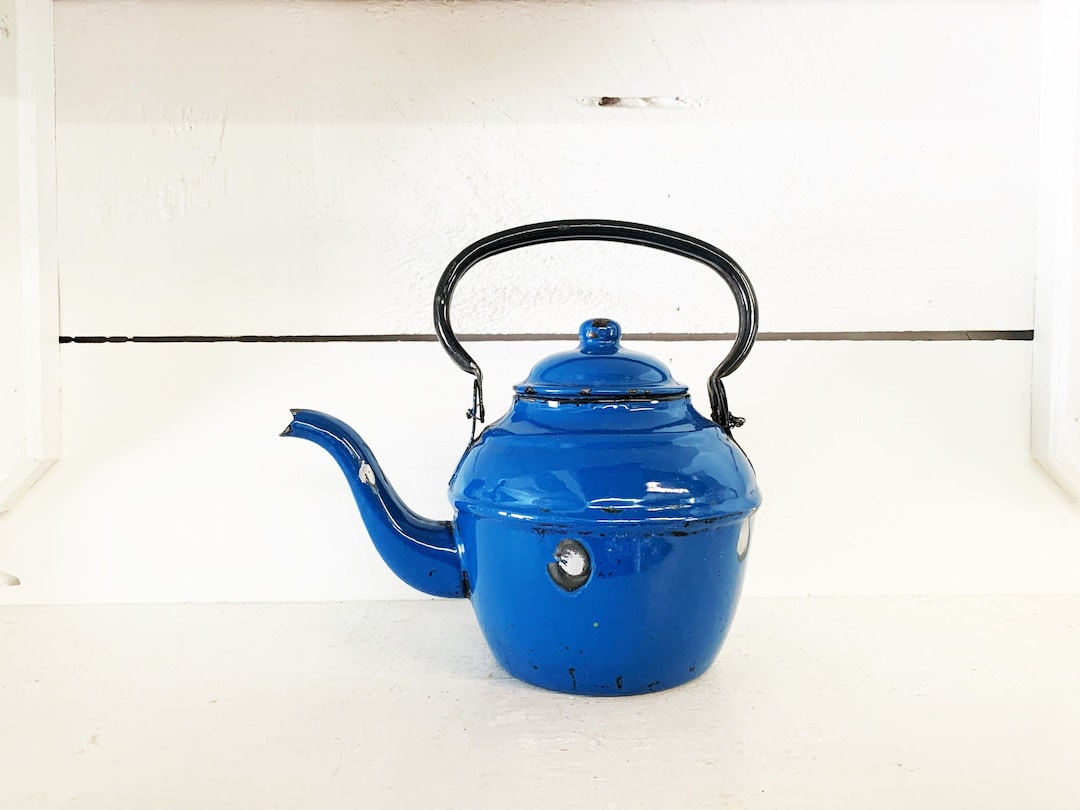The image is a close-up of an older style, large blue ceramic tea kettle with an elevated black metal handle. The spout, which faces to the left, has a noticeable chip in the paint revealing a silver mark, and there are black scuff marks at the kettle's bottom indicating wear and age. The kettle also features a small round lid with a knob on top, both slightly chipped. It rests on an off-white, textured surface, contrasting with the white textured wall behind it. A slim black line, likely part of a countertop or backsplash, horizontally intersects the background just above the midpoint, and a small chunk appears to be missing from the top of the kettle, further emphasizing its old, well-used condition.